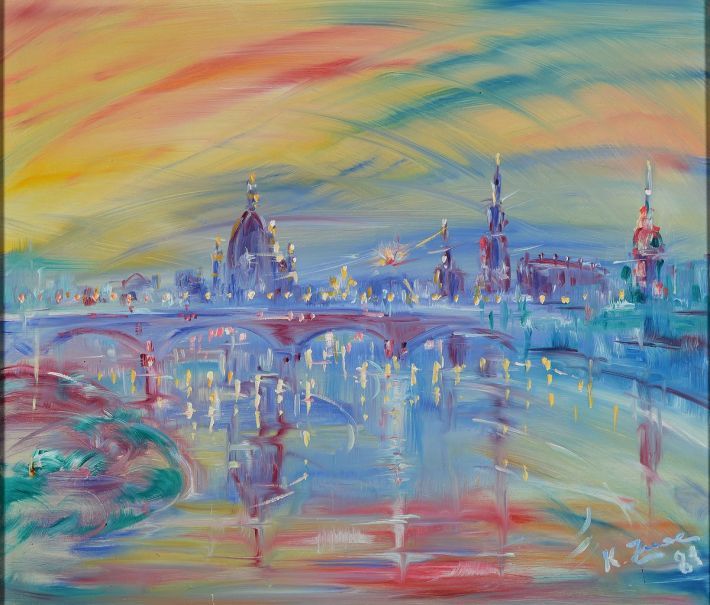The painting presents an impressionist view of a European city, rendered in a vibrant and abstract watercolor or possibly acrylic style. Dominated by light pastel hues and large brushstrokes, the image depicts a serene scene centered around a reflective body of water, which mirrors an array of softly blurred lights and a spectrum of colors including blues, yellows, reds, whites, and greens. In the foreground, there is a bridge adorned with multiple lights creating an almost festive atmosphere. The reflection in the watery surface suggests both the play of light and perhaps the vibrant mood surrounding an event like the 4th of July, enhancing the sense of celebration. In the background stand several tall buildings, painted mainly in shades of violet and lavender, although not reaching skyscraper heights. The sky above is a mesmerizing blend of orange, red, blue, green, and purple hues, evoking a late evening or twilight ambiance. The painting is signed in the lower right-hand corner, where the name appears to begin with a "K," followed by indistinct letters, and is dated, possibly with the year '81 or '84.'